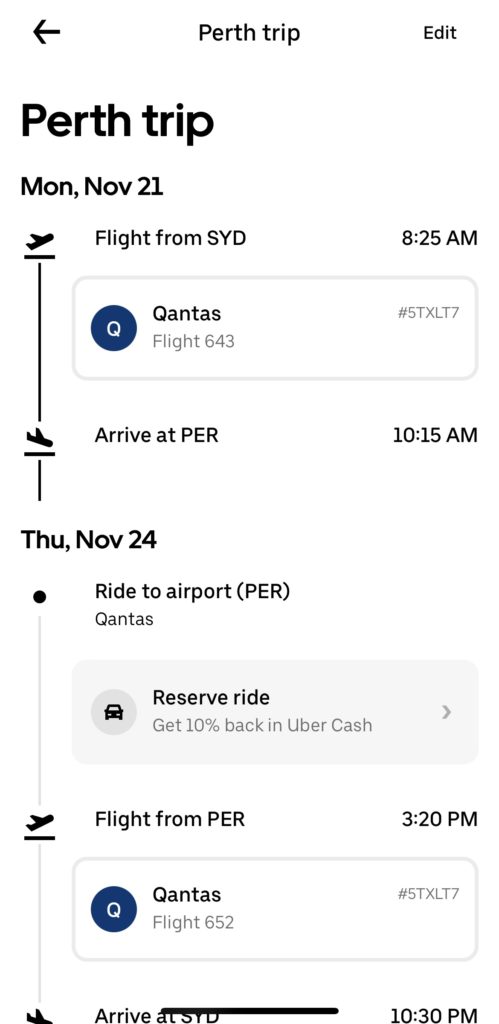Title: Detailed Itinerary for Perth Trip

Caption:
The image displays a comprehensive itinerary for a trip to Perth. At the top left, a black back arrow icon is visible, labeled "Perth Trip". Adjacent to it, there's an edit button. The title "Perth Trip" is prominently displayed below. The first entry on the itinerary is dated Monday, November 21st, beginning with a flight from Sydney (SYD) at 8:25 AM listed as Contos Flight 643. A circular icon with a white 'Q' on a blue background appears alongside the flight number 5TXLT7. The flight is scheduled to arrive in Perth at 10:15 AM.

The next section of the itinerary details the return trip on Thursday, November 24th. It starts with a "Ride to Airport (PER)" at an unspecified time, labeled again with the Contos brand, and offers a "Reserve Ride" option, promising 10% back in Uber Cash and displaying a black cab icon. The return flight from Perth (PER) is set to depart at 3:20 PM aboard Contos Flight 652, featuring the designation number 5TXLT7. The itinerary concludes with the arrival in Sydney (SYD) at 10:30 PM.

The various segments of the itinerary are interconnected by a dotted line, with all text presented in black on a white background, thereby ensuring clarity and ease of reading.